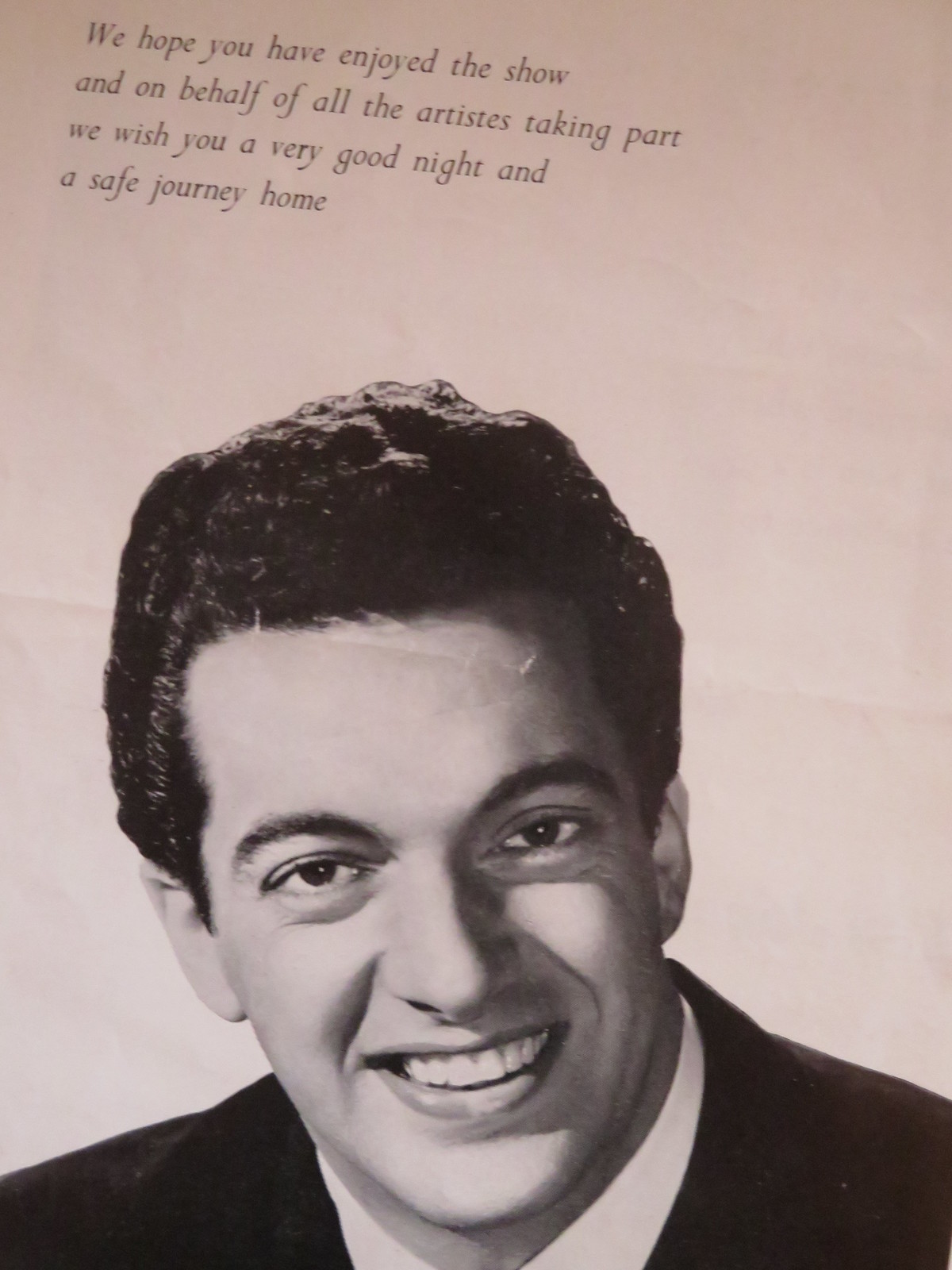The photograph is a vintage black-and-white headshot from a concert or performance, featuring a Caucasian man in his early to mid-thirties with short, curly black hair and thick, dark eyebrows. He is smiling broadly, showcasing his white teeth. Dressed in a black suit jacket with a white dress shirt underneath, he poses with a slight tilt in his body, making his left shoulder (our right) more prominent. Above him, in an italic script font on a peach background, is a message that reads: "We hope you have enjoyed the show and on behalf of all the artists taking part, we wish you a very good night and a safe journey home." The paper shows signs of age, including a noticeable crinkle, giving it an old, vintage feel.